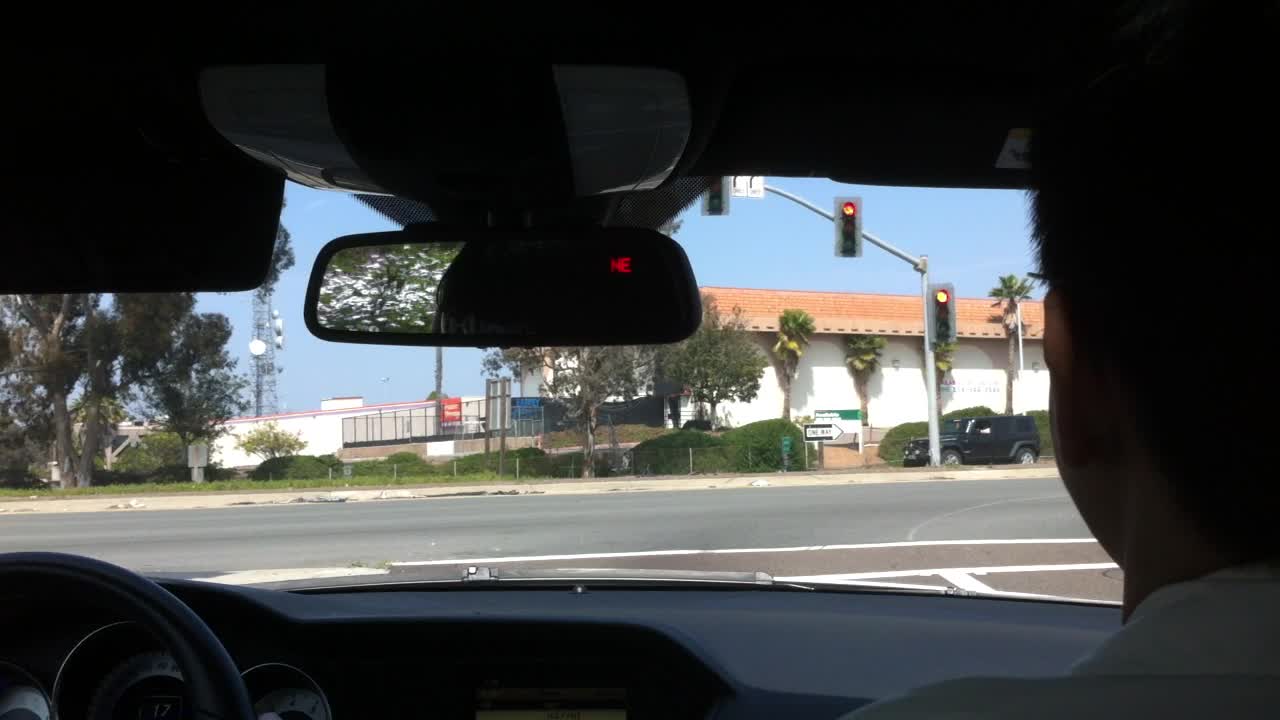The photograph is taken from the backseat of a car, capturing an interior view that includes the steering wheel, the instrument panel in the lower left corner, and the rearview mirror showing the driver’s forehead. The passenger in the front is wearing a white shirt. The car is stopped at a red light at an intersection. The light itself is mounted on a gray pole positioned on the right and overhead. The intersection features right-turn-only lanes, evidenced by road markings and a one-way street sign indicating a required right turn. 

In the distance on the left side, several palm trees suggest a tropical setting, while on the right side, there is a white building with a reddish-brown roof. A black Jeep Wrangler is crossing the intersection. Overall, the view through the windshield presents a detailed urban scene with a tropical backdrop.